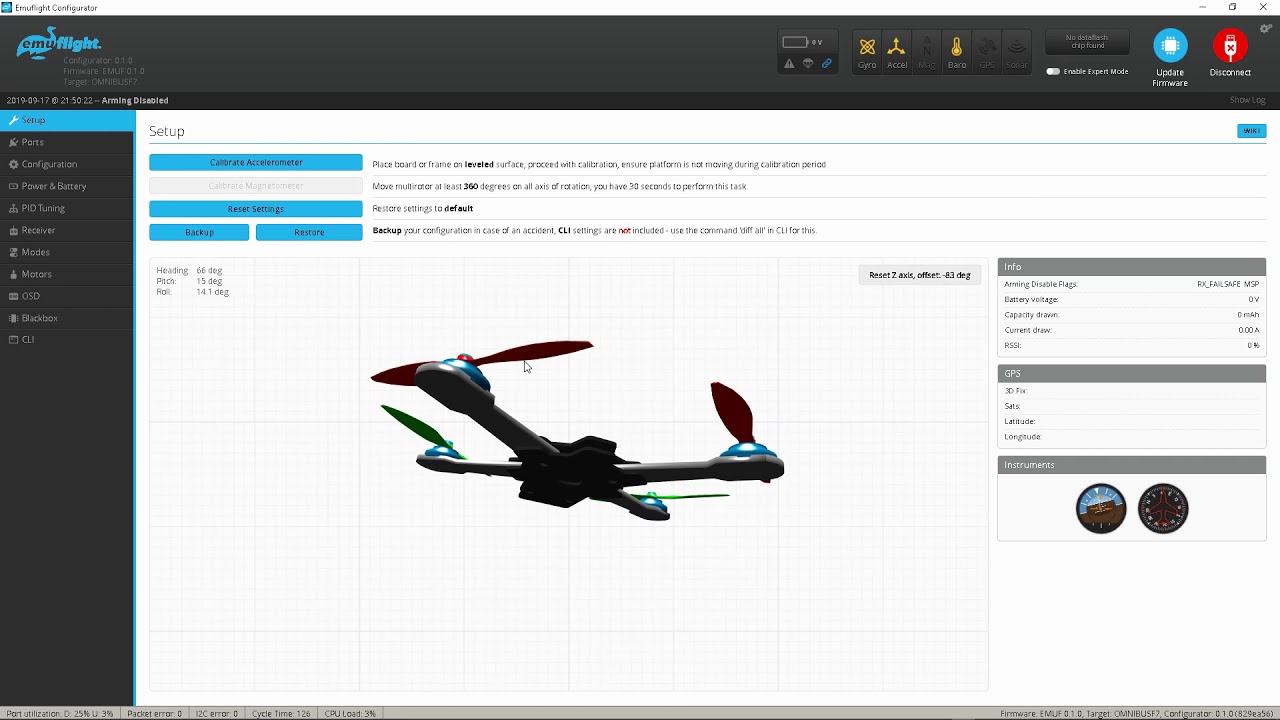The screenshot displays the EmuFlight software interface on a computer, used for configuring a drone. The page prominently features a detailed setup section, with a side menu on the left containing various sub-settings, the highlighted one being 'Setup'. The top banner showcases the EmuFlight logo—a blue duck—and provides firmware information.

On the right side of the top banner, several icons are shown, with three of them highlighted: 'Gyro' (gyrometer), 'Accel' (accelerometer), and 'Baro' (barometer). Nearby, large icons offer options to update the firmware and disconnect from the software.

The central section of the setup interface includes options such as 'Calibrate Accelerometer', along with fields displaying degree measurements for heading, pitch, and roll. Detailed instructions guide users on placing the board or frame on a level surface and moving the multirotor at least 360 degrees for calibration. 

The right side of the screen provides extensive information on battery voltage, capacity, and GPS data. An image of the specific drone being set up is also displayed, aiding in visual identification and configuration.